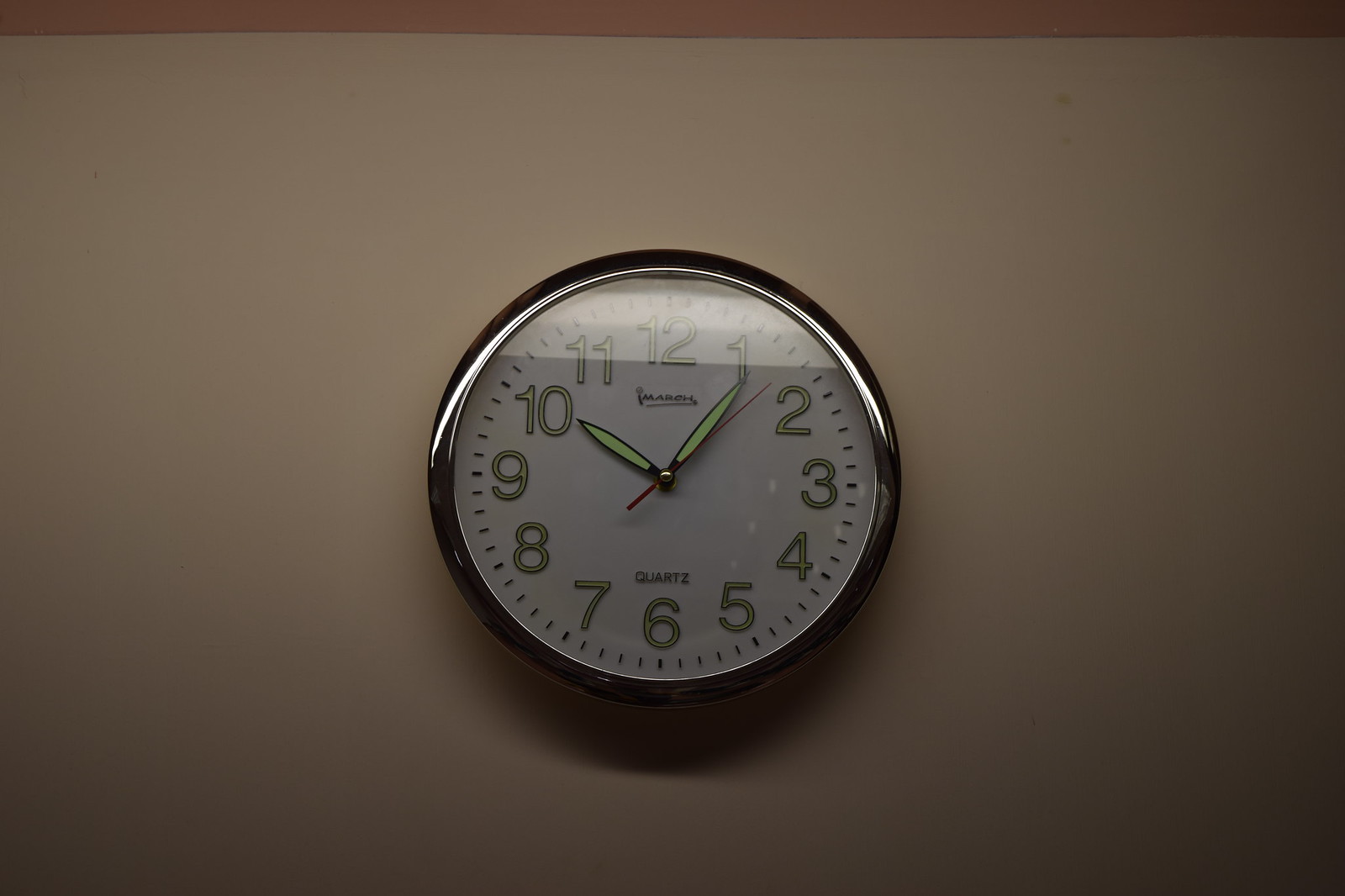The image showcases a round wall clock, hanging on a wall that appears to be painted in a khaki brownish color, accented with varying shades and some shadowing. The wall also exhibits a whitish surface near the top, with the edge of the ceiling displaying a tannish color. The clock itself has a shiny, reflective silver edge, which appears darker in the shadowed lower portion. The clock’s white face features numbers in a light yellowish color, boldly filled in yellow and outlined in black. The clock hands, which are designed to resemble plant leaves, are positioned to indicate that the time is 10:06. The hands are in a neon yellowish color, accentuated with a silver outline. Below these, the word "quartz" is printed above the 6. A reflection of a light source causes a slight distortion at the top, affecting the visibility of the 11 and 12. Additionally, it appears that "March" is written under the 12, though this is partially obscured by the shadowy background.